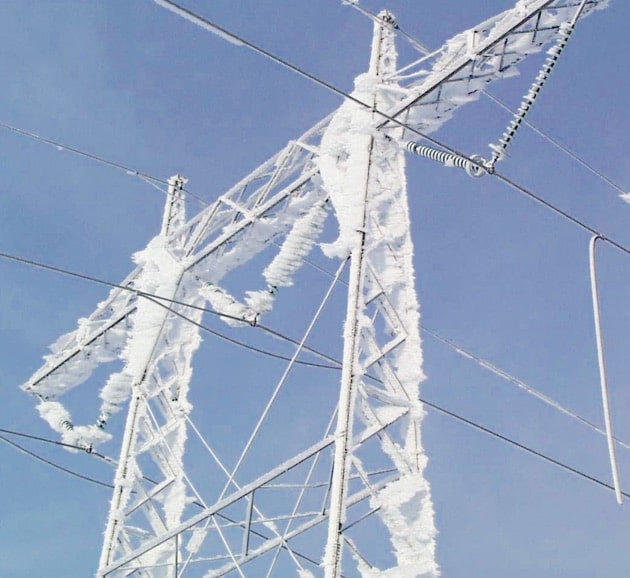The photograph captures an outdoor scene featuring tall, lattice-structured high-voltage electrical towers, prominently covered in ice and snow, set against a clear blue sky that transitions from light blue at the bottom left to a more saturated blue at the top right. The towers, seen from a low angle, stretch upwards and form a T-shape with horizontal crossbeams, supporting large diameter high wires with long insulators. The towers themselves are heavily frosted, giving a striking icy appearance, with less frost evident on the wires. The image, square in composition, vividly contrasts the clear daytime sky with the frosty, metallic structures, illustrating the harsh, wintry conditions enveloping the utilitarian architecture.